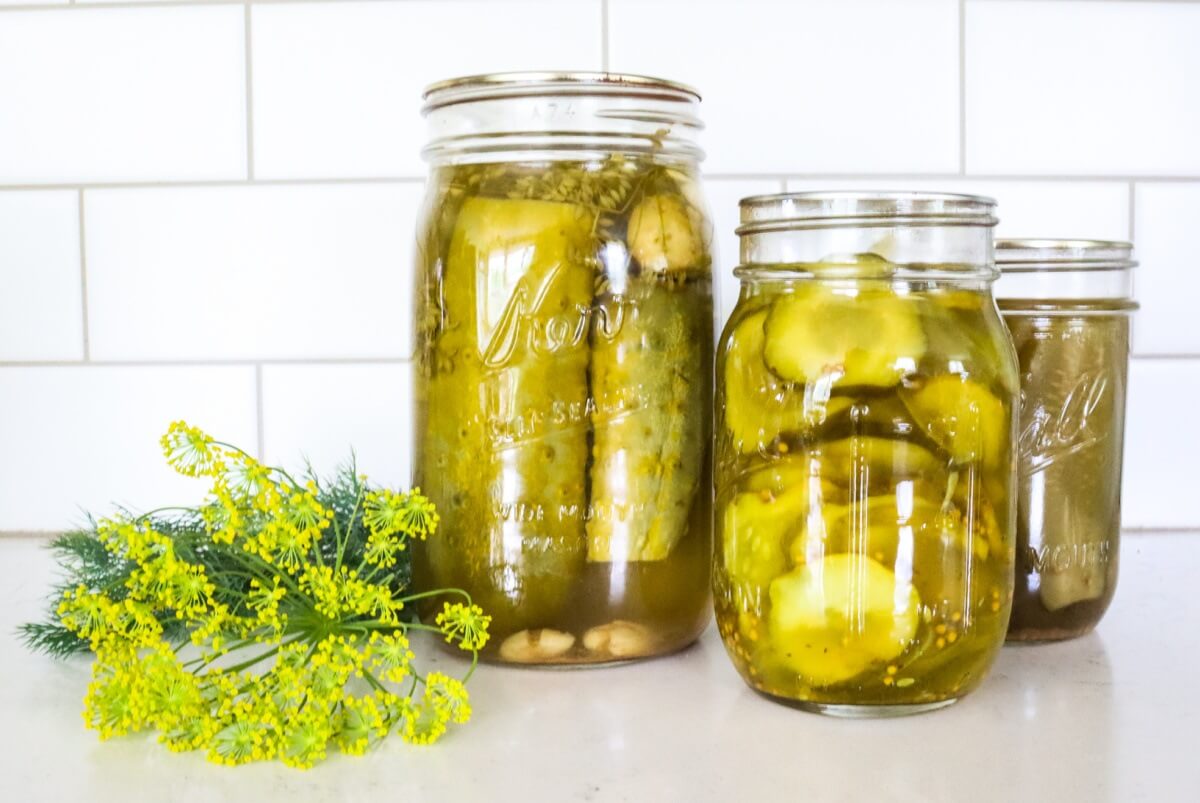The image is a detailed, high-resolution color photograph in landscape orientation, showcasing three glass jars filled with various types of homemade pickles. The jars are positioned side-by-side on a clear, white, glassy kitchen countertop. The background features smooth, white subway tiles with green grout, contributing to a clean and bright kitchen aesthetic.

The largest jar, situated in the center, is a clear Carr brand jar with a wide mouth and a silver lid. Inside are whole, vertically halved dill pickles with visible spices and two cloves of garlic at the bottom. To the right of this jar is a medium-sized canning jar filled with circular slices of pickled cucumbers surrounded by a flavorful broth. The smallest jar, partially obscured and placed to the far right, contains thin, vertical slices of dill pickles. 

Adding a touch of natural beauty to the scene, a sprig of yellowish dill with green stems lies to the left of the jars, resting on the countertop. The overall composition emphasizes the homemade and artisanal nature of the pickles, reinforced by the realistic, representational photographic style.